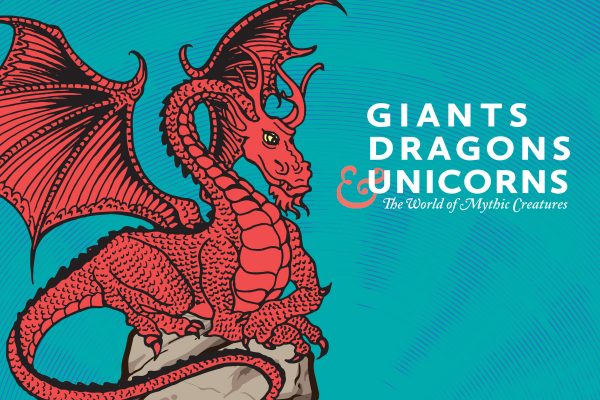The cartoon image, likely resembling a book cover, features a detailed dragon illustration set against a light blue background with scattered dark blue lines, giving it a textured look. On the right side, in distinctive white text, it reads "Giants, Dragons, and Unicorns" in bold, blocky letters, followed by "The World of Mythic Creatures" in a cursive-like font. Dominating the left side of the image is a meticulously drawn, big red dragon, outlined in black with intricate scaly details. The dragon sits on a gray rock, wrapping its long tail around it. The dragon has a yellow eye and red markings under its chin, with two visible teeth protruding from its closed mouth. It features two upward-pointing, red, spiky wings and crossed front arms with three visible talons on each foot. The dragon gazes towards the text, adding a dynamic and engaging visual element to the image.